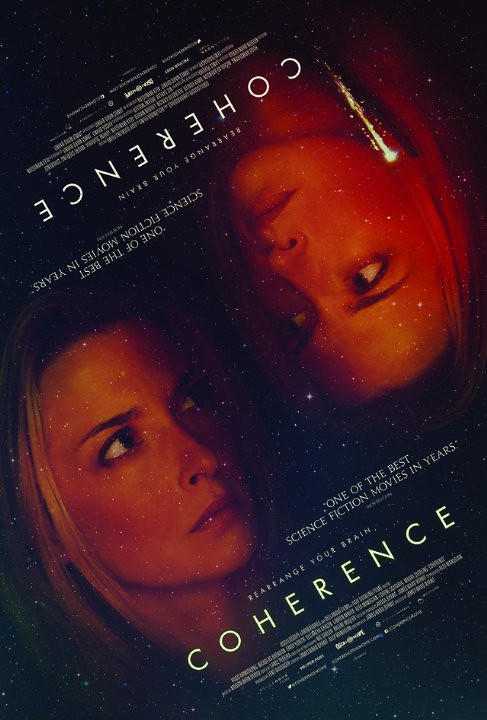The movie poster features a striking black background reminiscent of a night sky sprinkled with stars. Dominating the center of the poster is a mirrored image of a woman's face. The woman, who has blonde hair and a concerned expression, appears twice: once on the lower left looking to the right, and again on the upper right, flipped upside down, also looking to the right, creating a mirror-like effect. A flaming meteor descends in the bottom right corner, adding a dramatic touch. In white font, the poster proclaims, "One of the best science fiction movies in years," with the movie's title, "Coherence," prominently displayed beneath. The tagline "Rearrange Your Brain" suggests an intriguing, mind-bending experience. Fine print details the director and main cast, mirrored above and below the main imagery, ensuring the text is readable from any orientation.